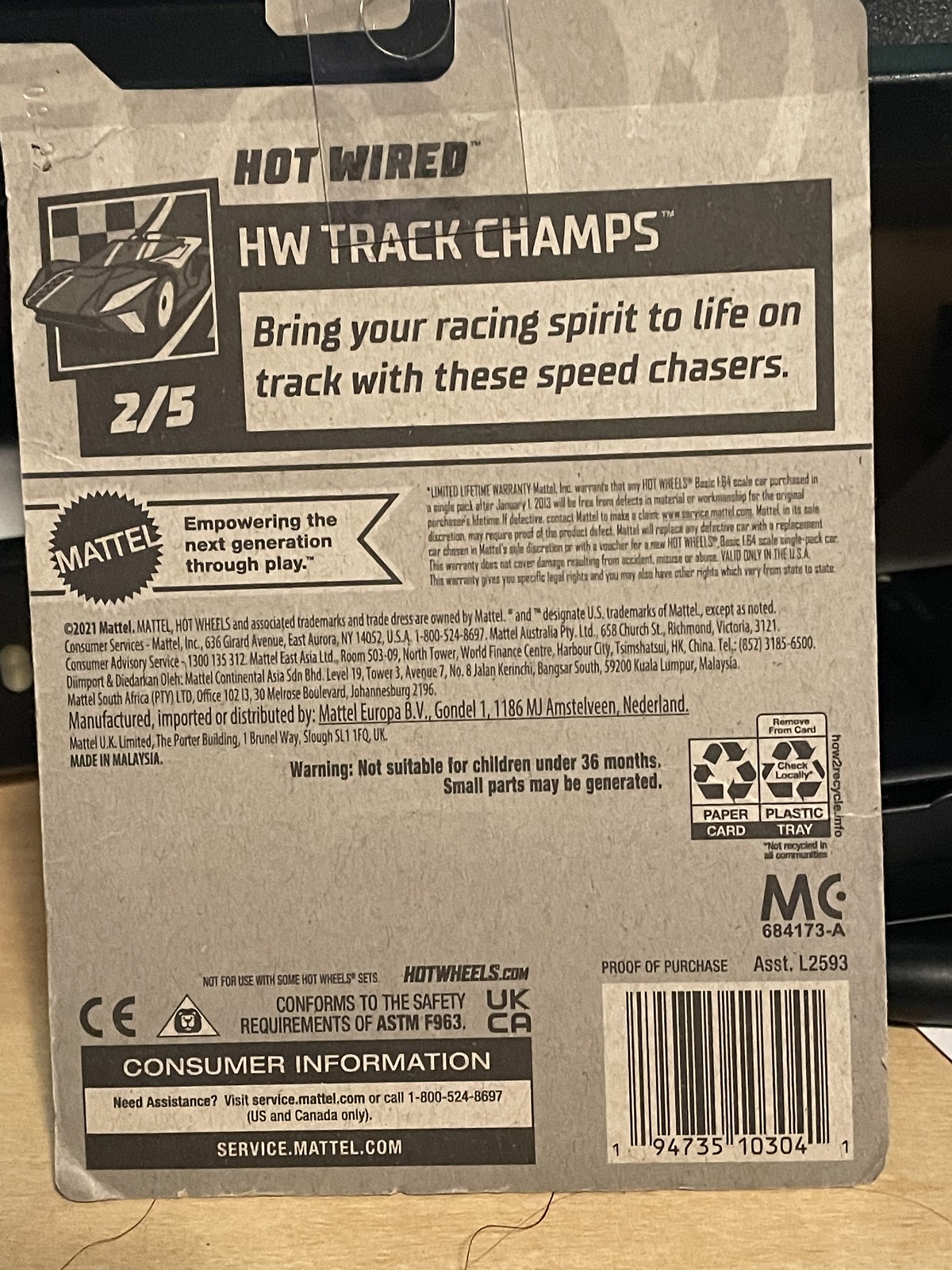The detailed description of this image depicts the back of a Hot Wheels toy packaging, made by Mattel. This cardboard backing features a plastic hanger attached at the top, likely because the original cardboard hanger wasn't sufficient for display. Dominating the top section is the image and artwork of a sports car, which appears dynamic as if jumping out of a square. Accompanying this artwork, text reads "Hot Wired HW Track Champs" and labels it as "2 out of 5" in its series. Below the image, a promotional line states, "Bring your racing spirit to life on track with these speed chasers." Further down, separated by a line, the iconic Mattel logo is displayed alongside the slogan, "Empowering the next generation through play." The bottom section is densely packed with requisite information and logos. This includes consumer information, a recycling logo, a barcode, an ISBN number, and warnings such as "Not suitable for children under 36 months," due to small parts. All of this is set against a deep gray and black background, with the texture and colors imparting a vintage feel to the packaging.